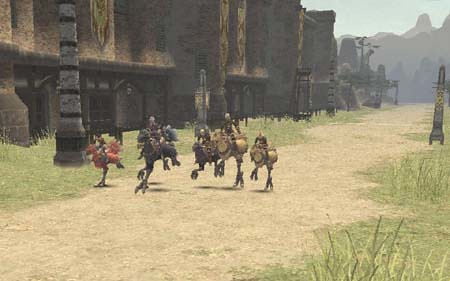This screenshot from a video game presents a dramatic scene along a lengthy, grassy path. The path, characterized by its shorter grass, stretches far into the distance, where dark, towering mountains loom ominously. On either side of the path, the grass grows tall and wild, adding to the natural, untamed atmosphere of the scene. Dominating the left side of the path is a foreboding, castle-like building, its dark, imposing presence casting a shadow over the landscape. Moving along the path towards the viewer are five fantastical creatures, resembling small dinosaurs. Each creature is ridden by a human, akin to equestrian riders. The composition of the scene, with its detailed environment and imaginative creatures, creates a vivid and immersive visual experience.